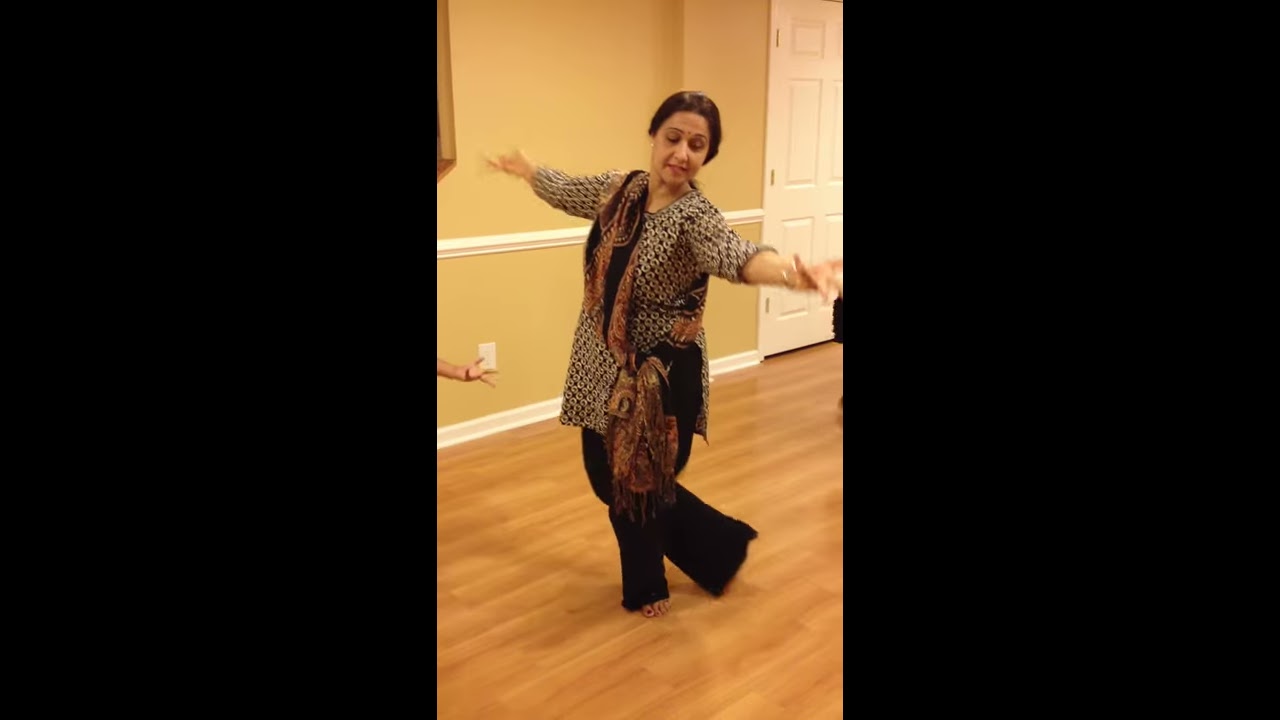The photograph features a woman dancing in a casual setting on a wooden floor. She has dark hair and is barefoot, wearing black pants and a long, printed tunic top with three-quarter sleeves. A striking feature of her attire is a long scarf, knotted at the side, cascading down to her knees. Her arms are outstretched, adding to the sense of motion, as one foot is poised in front while the other is placed behind her. The room features a beige wall with white trim and a white door visible to the right. A child's hand extends upward from the left side of the image, hinting at the presence of other participants, possibly fellow dancers, creating a lively, interactive scene. The image itself is displayed in a triptych format, with two outer black panels framing the central panel where the woman is captured in motion. A sense of joy and spontaneity pervades as she appears to be dancing for fun, perhaps engaging with the child nearby.